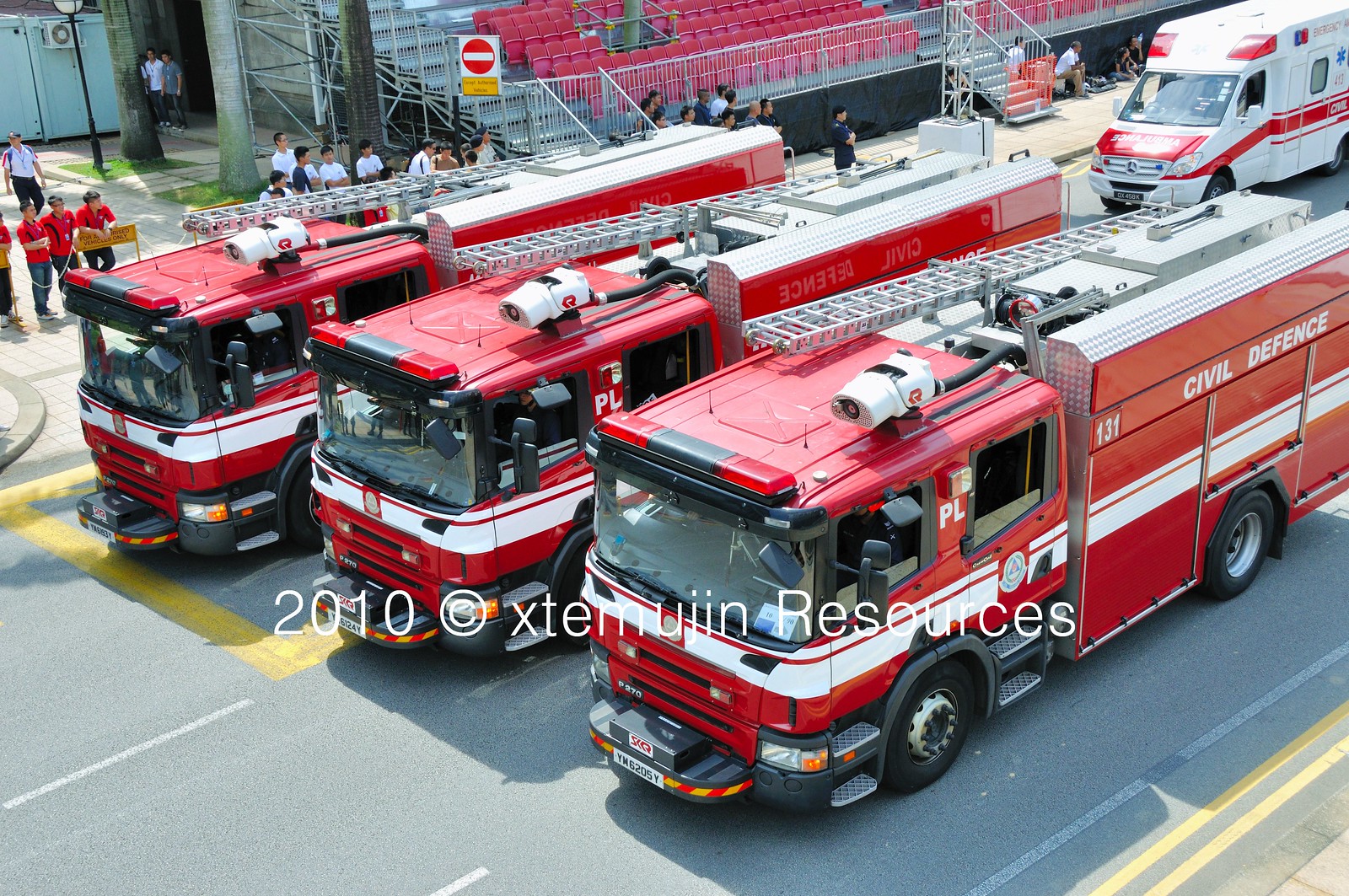This color photograph, taken in 2010 and attributed to Externum Resources (Xtemujin Resources), captures a scene at what appears to be a raceway or parade setup. The image prominently features three red Civil Defense fire trucks, each with two white stripes down the middle. These trucks are lined up in three lanes on a road, possibly preparing for a parade. The front truck has "Civil Defense" visibly written on its side, and each vehicle appears to be numbered. Positioned behind these trucks is a red and white ambulance, identifiable by the medical symbol on its side.

In the background, there are bleacher-style seats with red seating and silver metal stairs, suggesting a venue set up for spectators. A few people are seen lined up below the bleachers, observing the scene. The photograph's ambiance hints at a city setting, with a relatively small crowd possibly awaiting an event or parade.